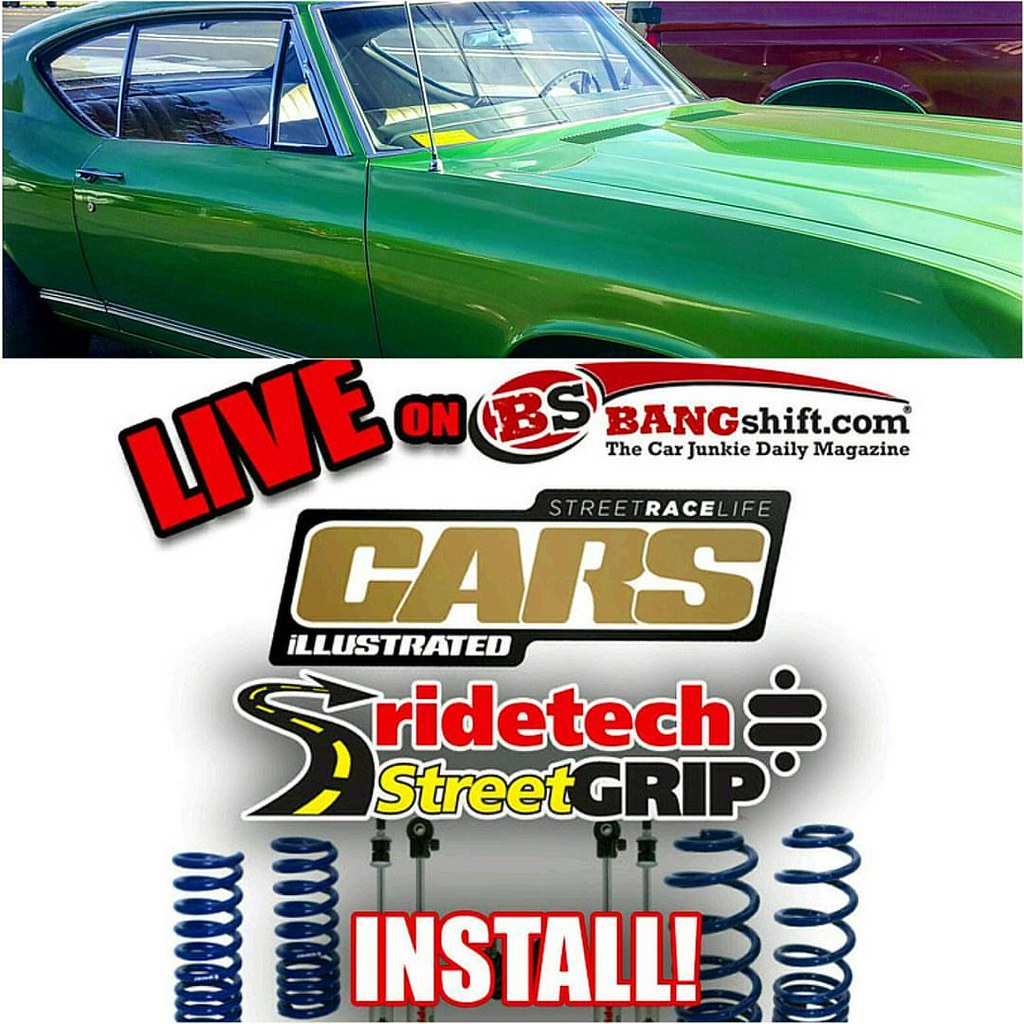The image features a top section showcasing an older, very clean, and shiny light green two-door car, presumably a Cadillac, set against the backdrop of a two-lane road visible through the windows. In the background, a purple car is also discernible. Below the car, there are several colorful text overlays and advertisements: 

- In bold red letters, "Live on BSBangShift.com" 
- Beneath that, it reads "The Car Junkie Daily Magazine"
- Following, in gold, it states "Cars Illustrated"
- Under that, in red text, it says "Ride Tech"
- In a combined black and yellow font, it reads "Street Grip"
- Finally, at the very bottom, outlined in red, it says "Install," with accompanying images of blue springs or coils next to the word.

The photograph, serving as an advertisement, balances vibrant colors and clear text positioning, making each element distinct and visually engaging.